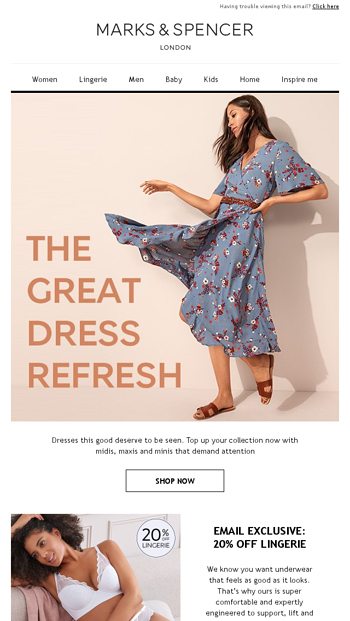The image depicts a sleek and stylish clothing website with a sophisticated header displaying the brand name "Marks and Spencer" prominently. Below the brand name, the location "London" is mentioned, suggesting a touch of British fashion influence. The website's navigation bar is featured higher up in the image, presenting various categories for an easy shopping experience: Women, Lingerie, Men, Baby, Kids, and Inspire Me.

Central to the image is a captivating promotional banner showcasing a vibrant scene where a woman exuberantly twirls in a wrap dress, conveying a sense of joy and freedom. Positioned at the bottom left of this banner is the promotional tagline: "The Great Dress Refresh." Following this eye-catching statement, there's an enticing description: "Dresses this good deserve to be seen. Top up your collection now with midis, maxis, and minis that demand attention." 

Encouraging immediate action, a bold and inviting "Shop Now" button is prominently displayed, urging viewers to explore and indulge in the latest dress collection. The overall impression is one of elegance and trendiness, compelling the shopper to dive into the offerings of Marks and Spencer.